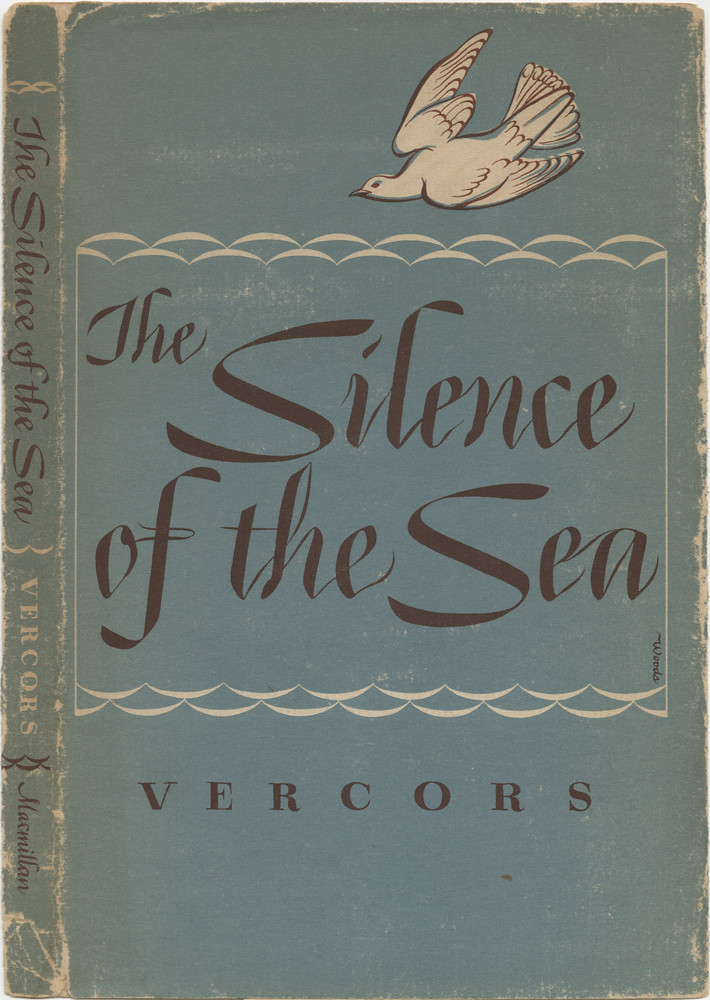The image displays a weathered and worn book cover that once was a bright baby blue, now faded with noticeable wear around the edges and spine. Dominating the cover is a serene white dove, positioned near the top right, its tail extending rightward and its face turned towards the center. The focal point of the cover is the title, "The Silence of the Sea," rendered in a distinctive semi-cursive black font, set amidst a surrounding pattern of white, wavy lines reminiscent of clouds or ocean waves. Below the title, the author's name, Vercors, is prominently displayed. This name also appears in white font on the spine of the book, emphasizing its importance. The book's publisher, Macmillan, is mentioned on the spine. The cover's condition reflects its age, with cracks, scratches, and discoloration revealing the book’s extensive use over time.